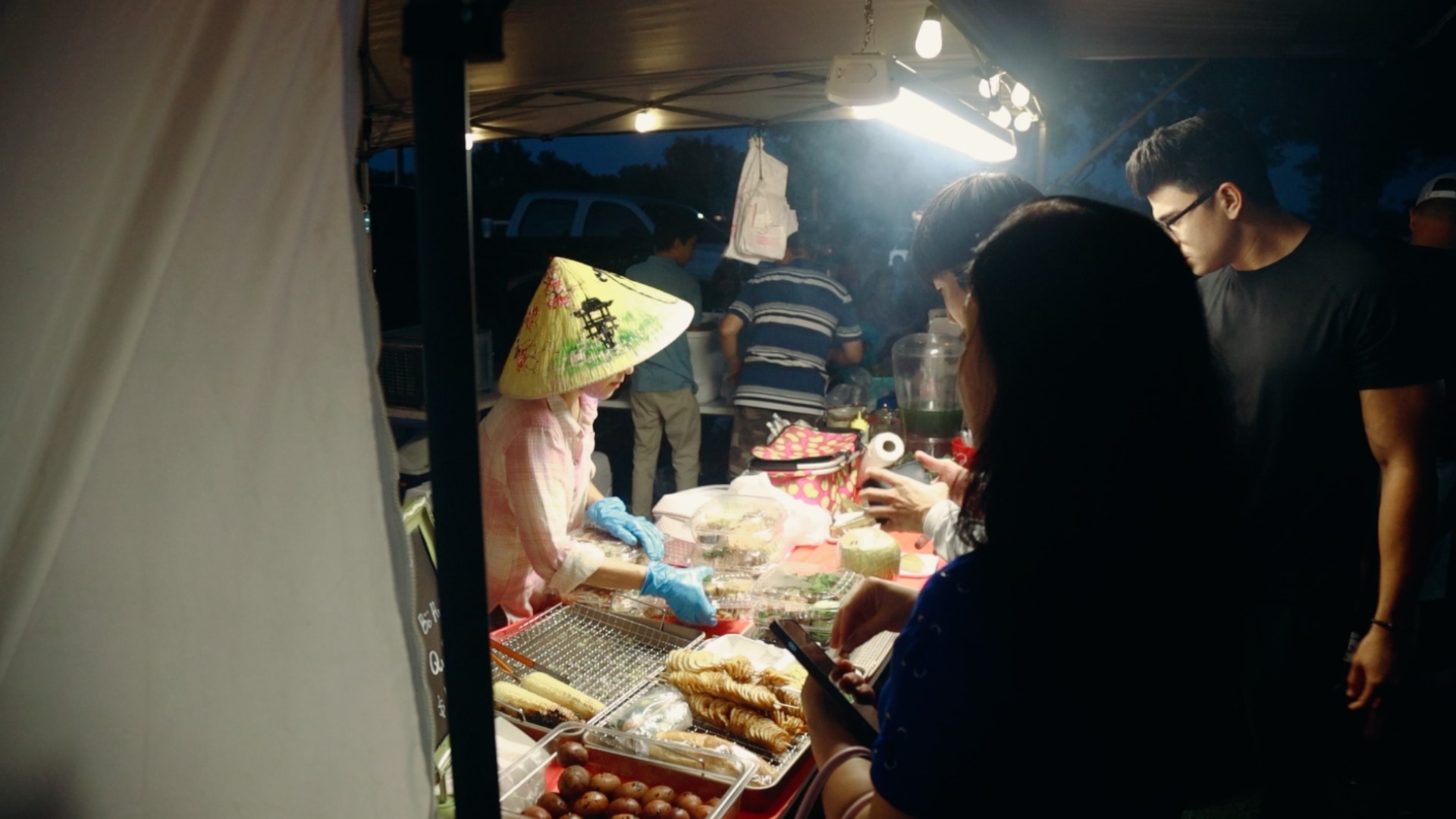This image captures the bustling scene of a nighttime street market, likely of Asian origin. Central to the image is a booth covered by a white tin canopy, illuminated by a bright, long fluorescent light hanging overhead. A woman, adorned in traditional attire including a pointed rice paddy hat and a pink blouse with her sleeves rolled up, is seen actively serving food. She dons blue latex gloves, indicating a focus on hygiene. Before her at the booth stands a group of customers: a man in a black t-shirt with glasses and short black hair, accompanied by two others whose faces are turned away, but black hair is visible. Behind the main booth, another table is set up with additional food items and people lined up, eager to order. The background suggests the market is set outdoors with a slightly dark sky and vehicles interspersed among a backdrop of trees, implying early nightfall. Though the specific location of this vibrant market is unclear, the scene vividly portrays an authentic, lively exchange centered around diverse food offerings.